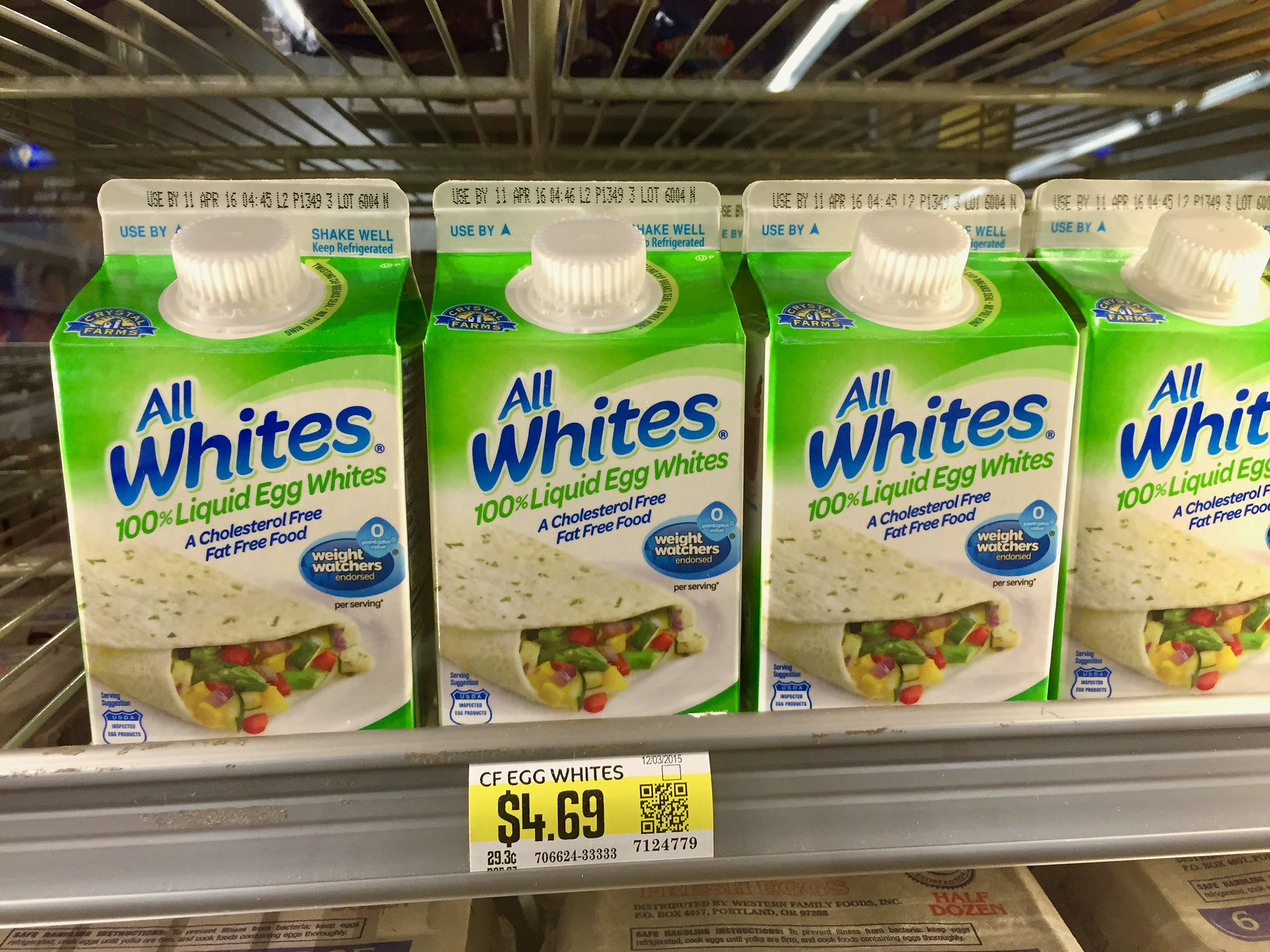The image features a close-up view of four pint-sized cartons of "All-Whites, 100% Liquid Egg Whites" sitting on a cooler shelf in a grocery store refrigerator. Each green and white cardboard carton has a white screw-top cap centered at the top. Prominently displayed on the front is a picture of a tortilla wrapped around a colorful mix of vegetables, including green, orange, and red pieces. The cartons are labeled with "All-Whites, 100% Liquid Egg Whites, Cholesterol-Free, Fat-Free Food" in blue text, and feature a Weight Watchers logo. Below the cartons, a price tag reads "CF egg whites, $4.69" along with a barcode. The expiration date on the cartons reads "Use by April 11th, 2016," and they include instructions to shake well and keep refrigerated. The image captures just a bit of the surrounding shelves, which are mostly empty except for some items potentially marked as a half dozen eggs.